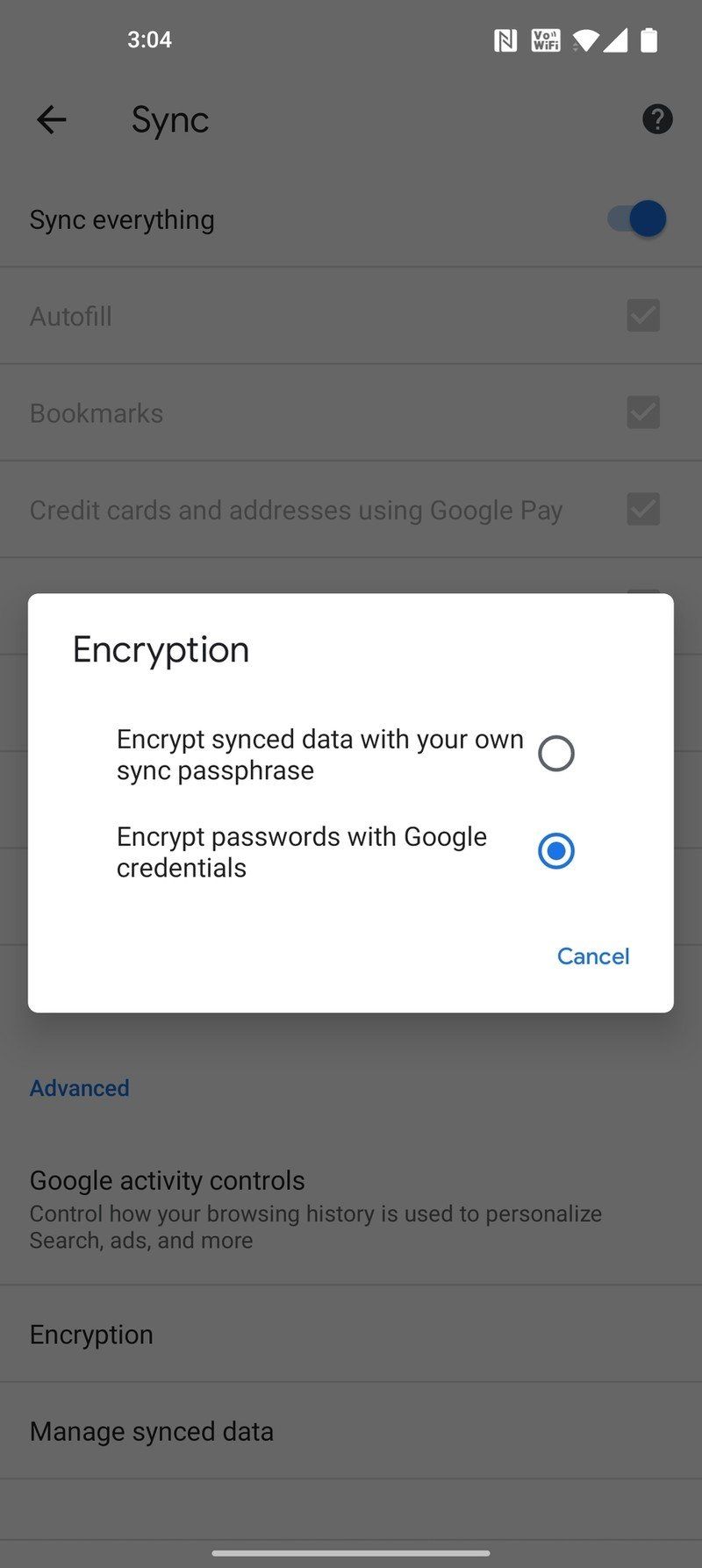This image is a screenshot taken from a smartphone display. The backdrop of the image is a dark gray, semi-transparent overlay, which slightly reveals the content behind it. At the forefront, a white dialog box is clear, holding a series of options concerning data encryption and synchronization.

At the top of the white box, bold black text reads "Encryption." Below this title, a message states: "Encrypt synced data with your own sync passphrase," accompanied by an unselected circular checkbox. Underneath this, another option reads: "Encrypt passwords with Google credentials," accompanied by a blue, fully selected circular checkbox.

Towards the bottom of the white dialog box, the word "Cancel" appears in light blue text, positioned on the left side, while "OK" is highlighted in bold blue text on the right.

The content displayed behind the white box pertains to synchronization settings. The title "Sync everything" is evident, with switches indicating the following options are enabled: "Autofill," "Bookmarks," "Credit cards and addresses using Chrome Pay," each marked with a check. Partially visible at the bottom of the image, and beneath the white dialog box, there are blue texts indicating further options: "Advanced," "Google activity controls," "Encryption," and "Manage synced data."

The screenshot captures a detailed view of the synchronization and encryption settings on a mobile device, showing user-selected options and available configurations for managing synced data and its security.